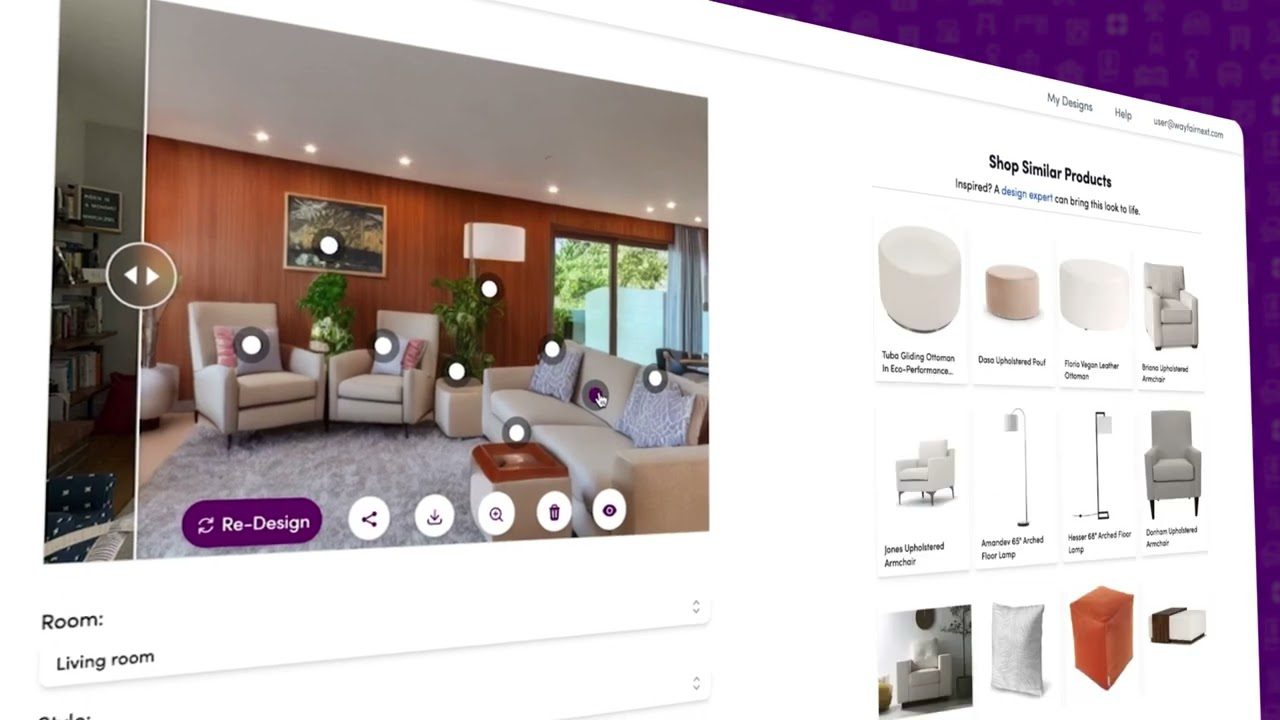The image is a detailed graphical representation, likely a screenshot or concept design of an interior design website or app. The visualization is presented with a 3D perspective, placed against a purple background and slightly rotated, providing a dynamic view that resembles an actual model rather than a flat screen.

In the depicted layout, the background is prominently visible on the upper right and far right edges. The focal point of the image is a stylish living room situated on the far left. This living space features a white ceiling, a light-colored area rug, and various pieces of white furniture, including a sofa, two armchairs, and what appears to be a footstool. The room also has a door leading to the outside, wood-paneled walls in a darker, cherry-wood-like finish, and multiple light sources, including ceiling lights and a floor lamp. Enhancing the room's ambiance are potted plants and a painting or graphical design on the wall.

Each furniture piece in the living room has small white dots on them, indicating interactive elements. These dots suggest that users can click on any furniture item, such as an armchair, to access more detailed information displayed on the right side of the screen. The right-hand section of the interface includes representations of each piece of furniture—like the floor lamp and chairs—where users can likely view specifics.

At the bottom of the living room image, a functional control panel with multiple buttons is visible. These include a purple button labeled "Redesign," along with options for sharing, downloading, expanding or zooming, deleting, and another button with an eye icon for additional functionality. Underneath the living room image, there is a label stating "Room" followed by "Living Room" and an adjacent dropdown menu, hinting at navigational options to view different rooms or scenes.

Overall, this image illustrates a sophisticated interior design mock-up for a website or app, providing users with an interactive experience to explore, customize, and gather information about various design elements within a room.